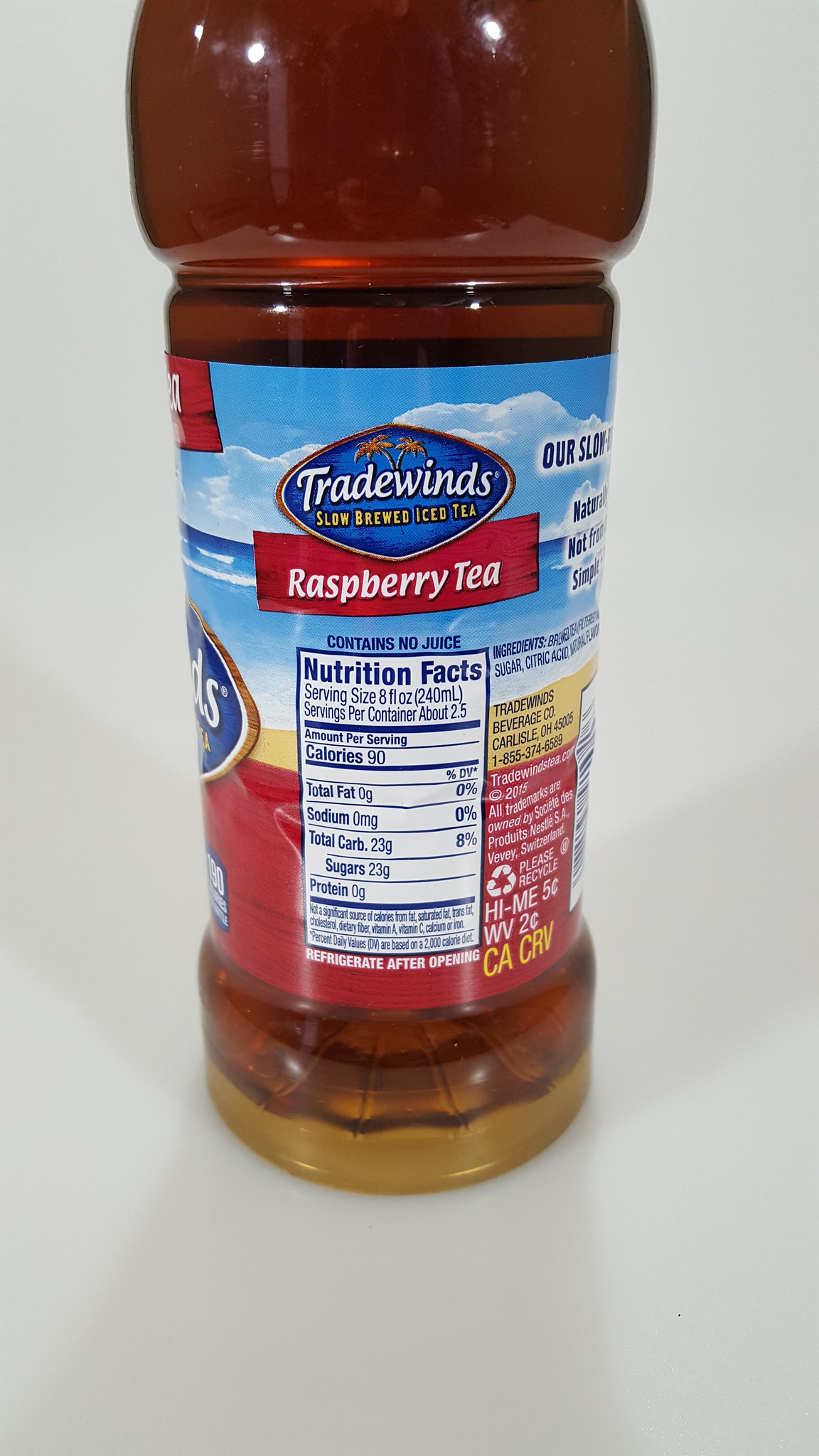A photograph of a bottle of raspberry iced tea shows a vivid red liquid inside the transparent container. The bottle reflects light from the top, enhancing its vibrant appearance. In the middle of the bottle, there's a detailed label featuring a wide blue circle decorated with palm trees at the top. The center of the circle prominently displays the brand name "NYTEX Tradewinds". Below this, in bold yellow text, it reads "Slow Brewed Iced Tea". Further down, a large red rectangle with white text proclaims "Raspberry Tea."

The lower part of the bottle contains a Nutrition Facts panel, stating the serving size as 8 oz (240 milliliters) and indicating approximately 2.5 servings per container. It lists the calorie count as 90 per serving, with 0.9 grams of total fat, 12 milligrams of sodium, and 4.2 grams of sugar. The label also instructs to refrigerate the bottle after opening. Additionally, it includes the ingredients and the manufacturer's name, "Tradewinds Beverage Co."

Towards the bottom, a recycling symbol is present alongside the refund values: "HI-ME 5¢," "WB 2¢," and "CA CRV," emphasizing the bottle’s recyclability in various regions.